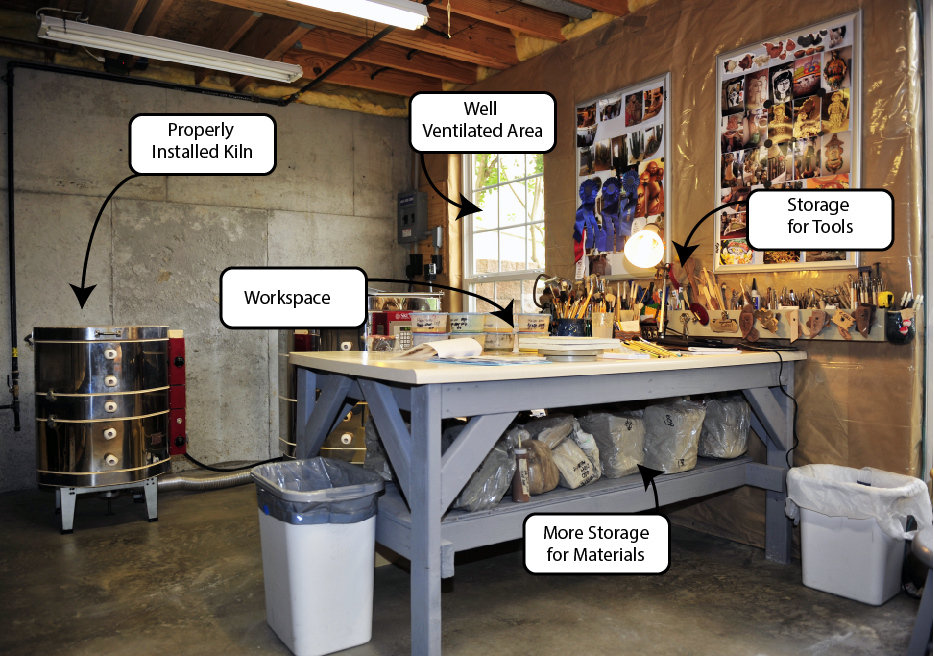The photograph captures a detailed view of an unfinished clay studio inside a garage or shed-like structure. The ceiling features exposed beams and tube lighting, while the floor is polished stone. The room's unfinished look is enhanced by bare concrete walls. Central to the image is a large, gray farmhouse-style workbench with shelving underneath, loaded with various supplies, including bags of clay, designated with a label reading "more storage for materials." Additional labels populate the image: "workspace" points to the table's surface, filled with craft supplies such as pencils and sculpting tools. On the side wall, a collection of paintbrushes and other tools are marked "storage for tools," stored in various cubbies. A significant feature is a shiny, silver kiln in the background with the caption "properly installed kiln." Flanking one wall is a window labeled "well-ventilated area." The studio is decorated with two posters depicting clay creations and has two trash cans situated on either side. Text bubbles with black borders and arrows punctuate the image, emphasizing the different sections of this highly organized creative space.